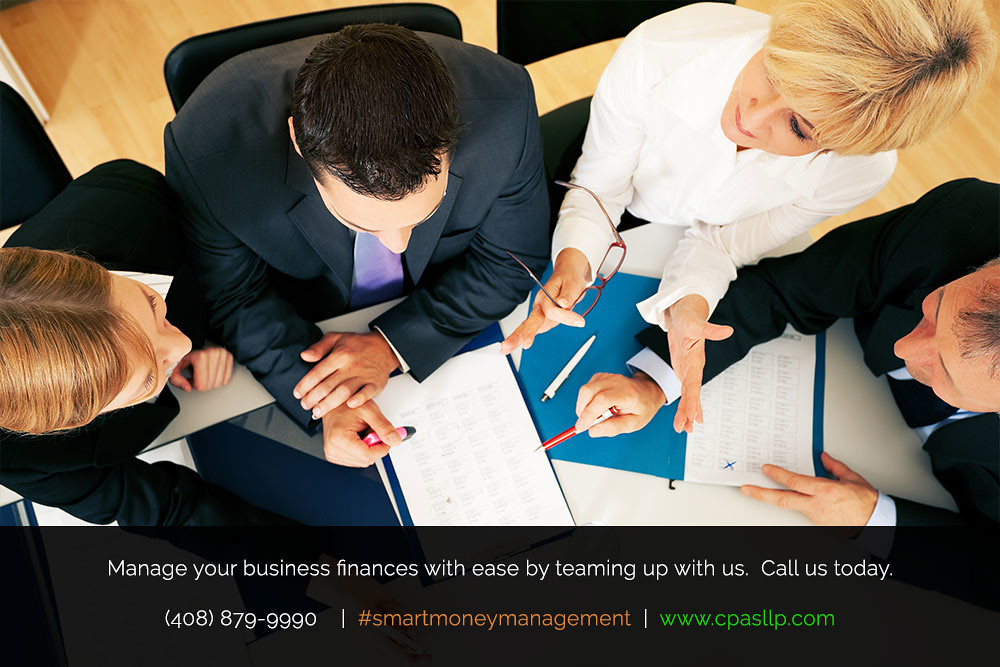This horizontally aligned rectangular image captures a bird's eye view of a business meeting in progress, used as an advertisement for smart money management. The photo focuses on the tops of the heads of four individuals engaged in discussing a report at a white desk. Positioned around the table, starting from the left, are a partially visible individual of indeterminate gender, followed by a man in the middle left wearing a navy blue suit with a light purple tie and holding a pen in his right hand. Next to him is a woman in a long-sleeve white blouse, with short blonde hair, holding reading glasses in her right hand. On the far right, another man is visible, holding a red pen in his right hand, with papers and a blue folder featuring an 'X' on the desk before them. The advertisement's text at the bottom reads, "Manage your business finances with ease by teaming up with us. Call us today," followed by the phone number 408-879-9990 in white print. The tagline "hashtag smart money management" appears in orange, and the website www.cpasllp.com is displayed in green to the right.